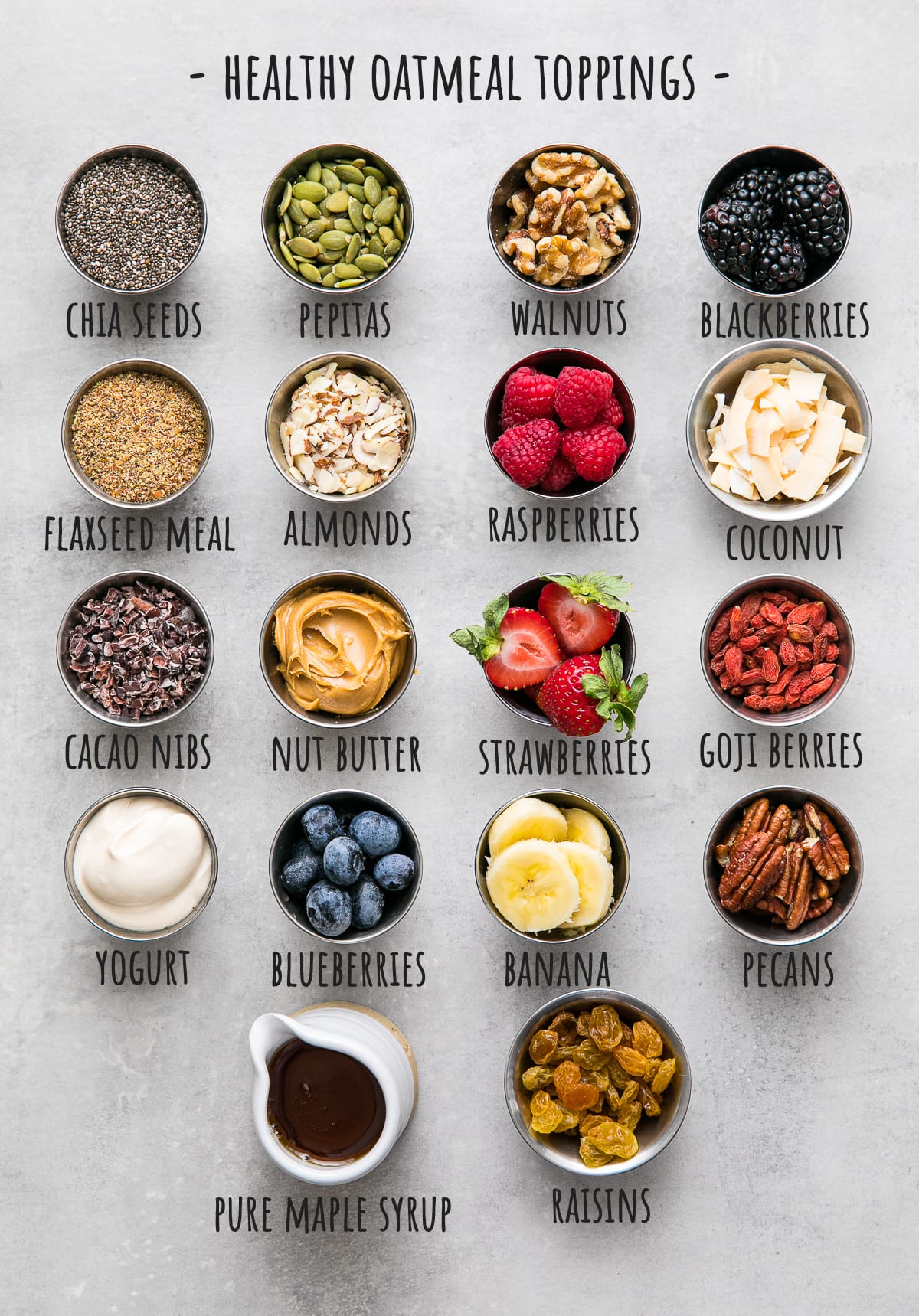This poster, titled "HEALTHY OATMEAL TOPPINGS" in bold black all-caps at the top center, features a detailed layout of 18 different nutritious ingredients in small, circular silver bowls. Each bowl displays a different topping, with the name of the topping labeled directly below it. The poster's background is a neutral gray, which contrasts with the vibrant assortment of toppings ranging in color from grays and greens to whites, reds, and blues.

In the topmost row, the bowls contain chia seeds, pepitas, walnuts, and blackberries. The second row presents flaxseed meal, almonds, raspberries, and coconut. The third row includes cacao nibs, nut butter, strawberries, and goji berries. In the fourth row, the bowls are filled with yogurt, blueberries, banana slices, and pecans. The bottom row features a small pitcher of pure maple syrup and a bowl of golden raisins.

The toppings are vividly colored, contributing to the poster's visually appealing arrangement. The blueberries are a rich blue, the bananas are neatly sliced, the pecans are a warm medium brown, yogurt is a clean white, and the goji berries have a distinct pinkish hue. This colorful and diverse array of healthy toppings makes for an interesting and inviting selection to enhance any oatmeal dish.